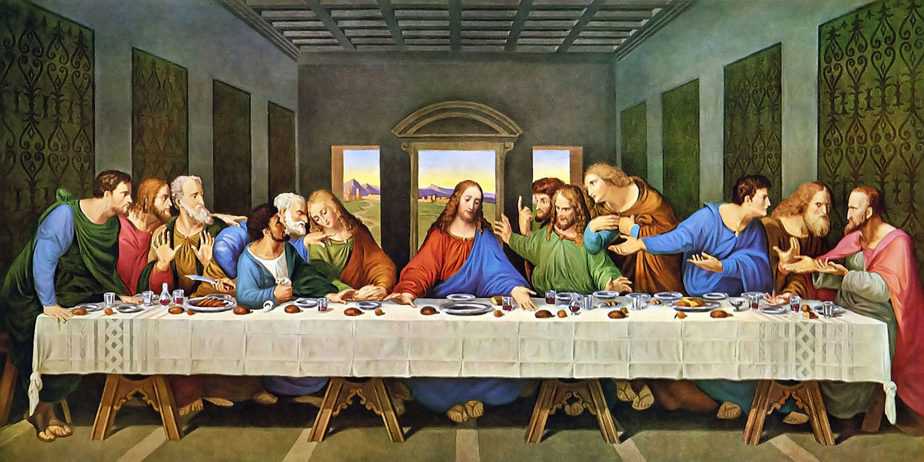This painting of the famous Last Supper portrays Jesus at the center of a large table, adorned with a white tablecloth and situated on wooden sawhorses. Jesus is dressed in a red and blue robe, and his serene hands rest on the table. The scene captures various expressions and interactions among the disciples, who flank Jesus on both sides, wearing colorful robes. Some are engaged in conversation, while others appear to be arguing, with a few pointing towards Jesus and looking at him. In the background, the room features walls with intricate patterns and large glass windows that reveal an outside view of a bright blue sky with hints of yellow and distant rolling hills. On the table, there are plates, food, and wine glasses. The overall artwork stands out with its vibrant colors and detailed depiction, giving it a sense of modern enhancement compared to traditional renditions, and evokes a strong religious atmosphere typical of such sacred themes.